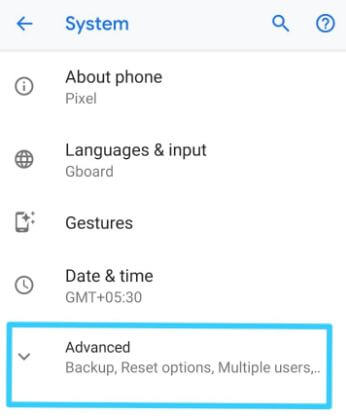Screenshot depicting a predominantly white interface with various blue and aqua elements. At the top, a blue arrow points left towards the words "System" and "Search." Adjacent to these, a blue circle encompasses a question mark symbol. Below it, there's a blue circled eye icon labeled "About Phone," indicating Pixel devices. Additionally, there's a globe icon labeled "Languages and Input," which specifies "Gboard." Further down, an icon of a phone with a plus symbol next to it is labeled "Gestures." Following this, a clock icon is paired with "Date and Time," showing "GMT +05:30." The final section shows an aqua-colored box with a downward-pointing arrow, labeled "Advanced." This includes sub-options: "Backup," "Reset Options," and "Multiple Users." The screenshot cuts off at this point, encompassing a detailed view of a device's settings menu.